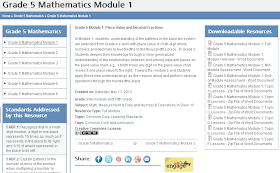The image features a compact and detailed layout, beginning with a small, light gray rectangle at the top. This rectangle contains the text "Grade 5, Mathematics, Module 1." Directly below, a larger blue rectangle is present, though the white text within it is too small to be deciphered at this resolution. On the left-hand side of the image, another blue rectangle with white writing is positioned.

Further down the layout, there are several gray-outlined rectangles, each containing a symbol on the left and accompanying text. Continuing, there's another blue rectangle featuring white writing, followed by some gray text beneath it. A vertical blue line is also observed, beside which gray text is written.

Towards the bottom of the image, a symbol is followed by more gray text and a cluster of possible social media icons. Additionally, a yellow rectangle with black and orange elements is identifiable. On the right-hand side, another blue rectangle with white writing can be seen, situated above an area densely packed with gray text and lines, possibly including numbers or symbols that are not discernible.